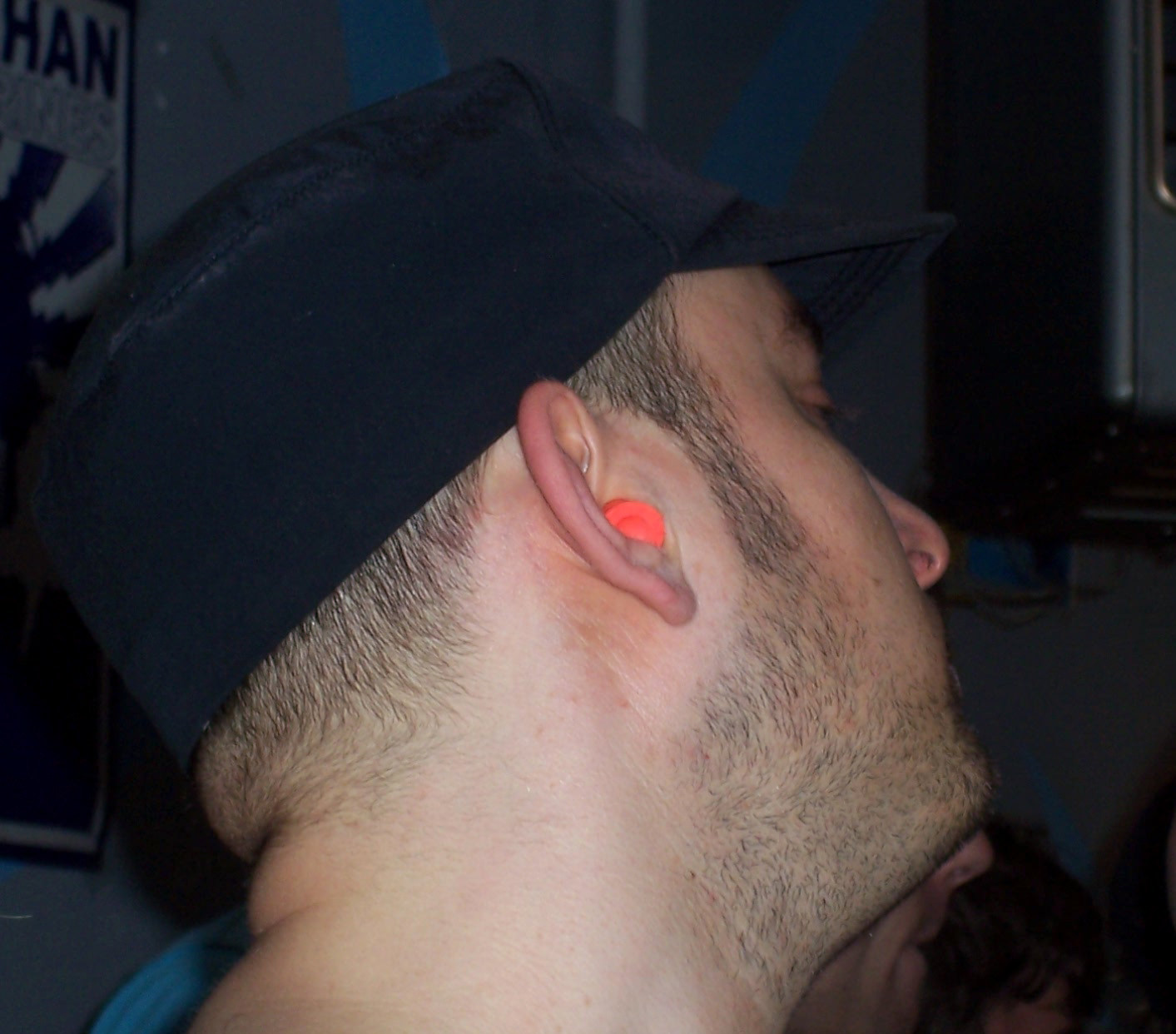The photograph is an indoor, color shot primarily showcasing the right-side profile of a white male, approximately 25 years old, against a dimly lit background that appears to be a room. The man is wearing a black military-style baseball cap, and has very short, closely-cropped hair with some strands peeking out from under his cap. He sports a scruffy beard that transitions from his short sideburns. An orange earplug is prominently visible in his right ear. The man is dressed in a blue shirt. The focus is on the three-quarter view of the back of his head, particularly emphasizing his right ear, nose, and eye. In the lower background, the faint profiles of two other individuals can be seen: one is a woman with round curly hair, and the other is a person, slightly more discernible, showing their nose, mouth, and cheek. The surrounding areas of the image are dark, accentuating the minimal lighting on the subjects.